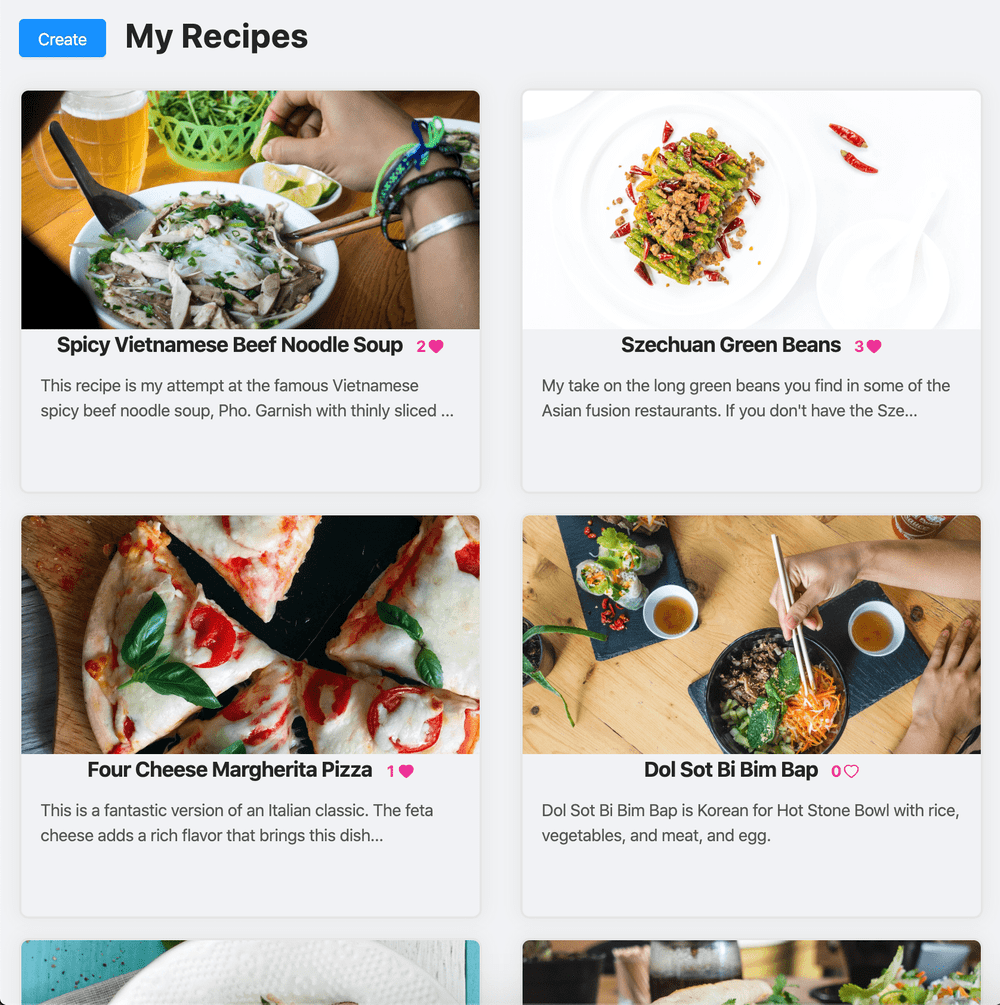A screenshot of a home page showcasing saved recipes is displayed. The main section is divided into rectangular tiles, each featuring an enticing image of a dish accompanied by its name in bold text. The highlighted recipes include Spiced Vietnamese Beef Noodle Soup, Szechuan Green Beans, Four Cheese Margherita Pizza, and Bibimbap. Each title is accompanied by an icon of a pink heart, likely indicating the number of users who have favorited or saved these recipes. While the top halves of two additional recipes can be seen, their titles and images are too obscured to be identifiable. On the left side, in a bolded blue font, is a button labeled "Create." At the top of this section, the words "My Recipes" are prominently displayed, indicating the personalized nature of this collection.